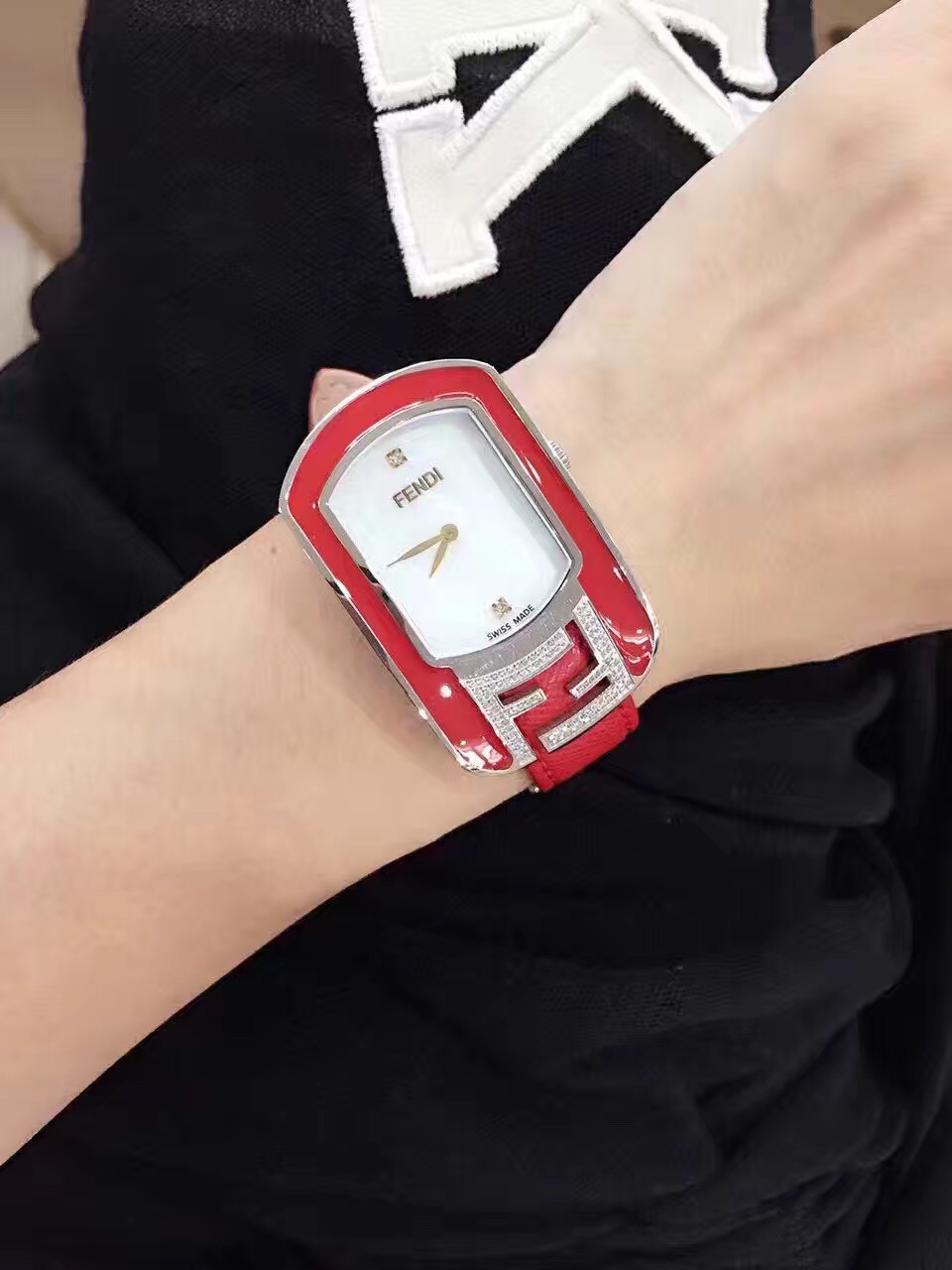A photo captures a Fendi wristwatch displayed prominently on a slender, fair-skinned wrist, likely belonging to a female. The watch's face is uniquely designed with an arched top and bottom, featuring elegant vertical lines. Gold hour and minute hands stand out against the backdrop, beneath which the Fendi logo is clearly visible. Additionally, some indistinct markings can be noticed below the logo. The sophisticated timepiece is complemented by a vibrant red leather strap, adorned with mirrored 'F' patterns that appear to be encrusted with diamond-like details. Due to the cropping of the image, only a portion of the wrist is visible, with the fingers out of the frame.